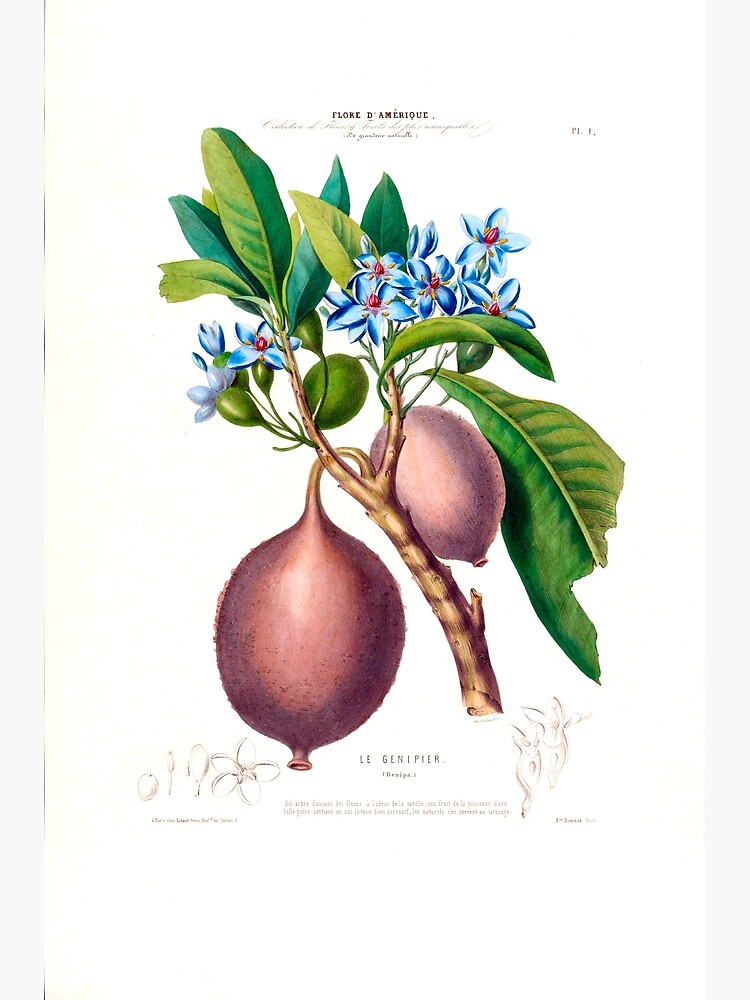This image appears to be a detailed botanical illustration from a book or textbook, depicting a plant with a central, light pink-to-maroon bulb or fruit, possibly a juniper berry. The artwork is richly colored and intricately drawn using pen and ink, featuring an array of colors such as green, yellow, blue, magenta, purple, tan, and bronze. The central bulb is attached to a brown twig, surrounded by a variety of blue flowers that exhibit a gradient from light to dark blue, with pink buds in their centers. Small olive-like buds connect these flowers to the twig. The foliage includes green and blue-green leaves of different sizes, each leaf elongated with a prominent vein running down the center.

At the top of the image, the faint and almost illegible text reads "Flor de Amérique," with a page marker noting it as "page one." Below the central illustration, faint sketches detail individual parts of the plant, including the bud, flower, and twig. Additional text, also quite faded, appears beneath these sketches but remains largely unreadable. The bottom of the image prominently displays the script "Les Genipères," suggesting the subject might involve juniper flora. Overall, this plate provides a systematic, visually appealing presentation typical of botanical volumes, aimed at carefully identifying and describing each component of the plant.